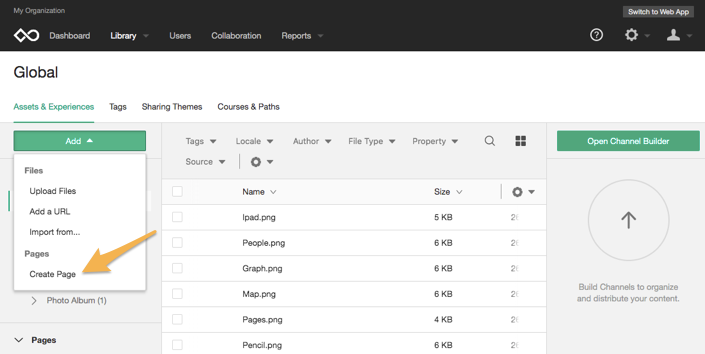The image depicts a web application interface for managing an organization's digital assets. At the very top left corner, there's the text "My Organization," while on the top right, there's an option to "Switch to Web App." Just below this is a logo, followed by a horizontal menu bar with the options: "Dashboard," "Library," "Users and Collaboration," and "Reports." To the far right of this menu bar, there are several icons: a question mark (help), a settings wheel, a down arrow, an image icon representing a person, and another down arrow.

Below this, the interface displays the word "Global" adjacent to another horizontal menu with options: "Assets and Experiences," "Tags," "Sharing Themes," and "Courses and Paths." Notably, "Assets and Experiences" is highlighted. Under this section are options for adding content: "Add Files," "Upload Files," "Add a URL," "Import from Pages," and "Create Page," with an indicator pointing to "Create Page."

To the right of this options box is another set of horizontal choices: "Tags," "Locale," "Author," "File Type," "Property," a magnifying glass icon for search, and four squares likely representing a menu.

Below that, there's a label "Source" followed by a settings icon and a list of selectable file categories. The categories listed are:
- Name: iPad.png, People.png, Graph.png, Map.png, Pages.png, Pencil.png
- Size: 5 KB, 6 KB, 6 KB, 6 KB, 4 KB, 6 KB

Further down, next to a "Settings" section with numbers that appear to begin with "2" (likely two-digit values), there's an actionable "Open Channel Builder" button. Beneath this button, a circle with an upward-pointing arrow and the phrase "Build channels to organize and distribute your content" invites users to engage in channel creation for content management.